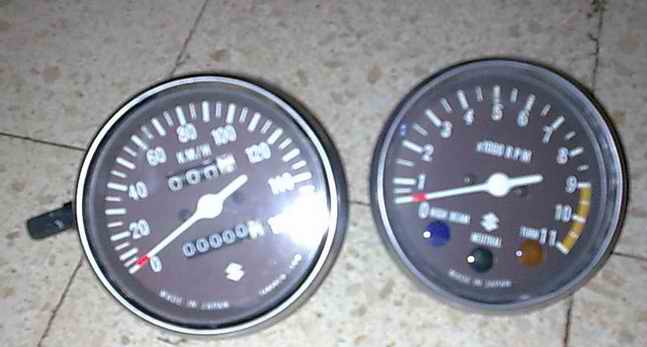In this landscape-oriented photograph, two unconnected pressure gauges are placed on a splotchy linoleum floor, which mimics the appearance of granite or rock and features noticeably dirty grout lines. The gauges are somewhat blurry, making it difficult to discern any specific wording or the manufacturer's name. 

The gauge on the left has a black casing and measures from 100 to 160, but its needle is resting at zero. The second gauge, also black, ranges from 1 to 11 and is likewise set at zero. This second gauge is equipped with three unlit buttons, colored blue, green, and orange, indicating potential functionality. The overall image conveys a sense of neglect, emphasized by the grime in the grout and the disconnection of the gauges from any system.